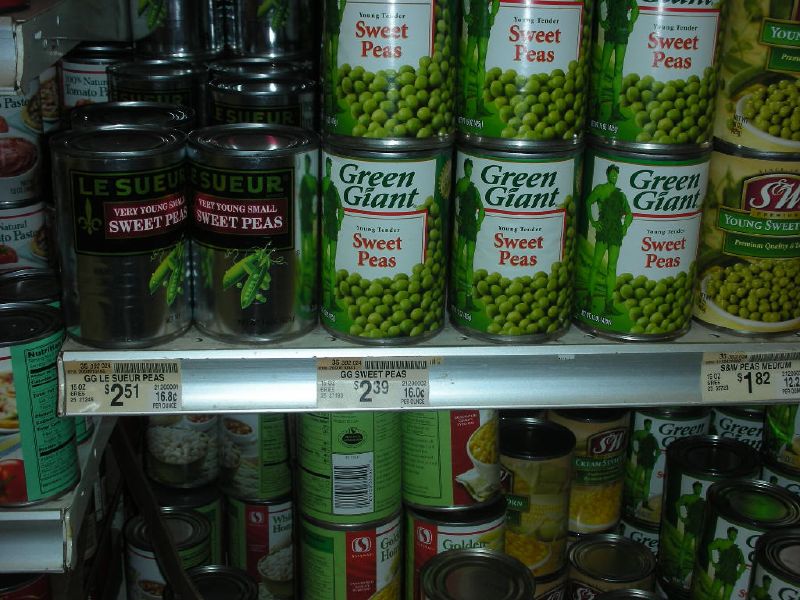The image captures a section of supermarket shelves stocked with various canned goods. At the top, an array of green peas in tins is prominently displayed, with the central portion featuring the recognizable Green Giant brand. On the left side of this top shelf, cans of sweet peas from the Le Sueur brand are arranged, while to the right, indistinguishable cans occupy the space. The shelf directly below presents a disorganized assortment of tins. Among them, a few Green Giant sweet corn cans can be discerned, though the majority of the cans are turned away, obscuring their labels from view. Towards the left edge of the second shelf, there appears to be a cluster of tins that might contain tinned tomatoes. Additionally, the edge of another shelf is visible on the left-hand side of the image, hinting at the broader context of the supermarket or shop setting.